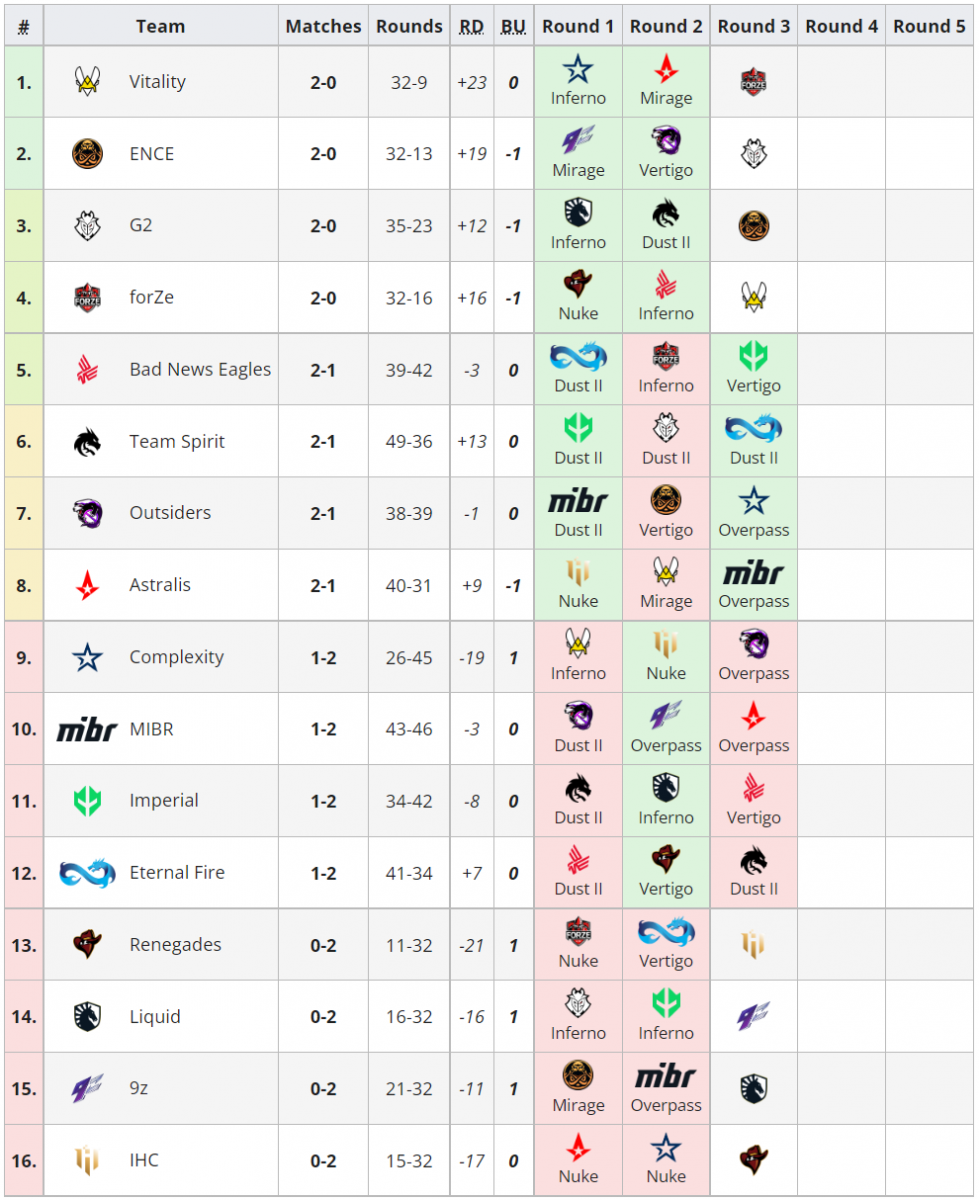**Detailed Description of the Tournament Progression Chart:**

The image is a comprehensive and colorful tournament progression chart divided into several sections.

1. **Header**:
   - The top section features a grey rectangle spanning the width, containing various labels and graphical elements.
   - On the right-hand side, there's a number sign (#) symbol.

2. **Teams and Matches**:
   - Underneath the header, the chart is structured by rows and columns.
   - The first column is labeled "Team" and lists the different teams along with their respective logos sequentially.
   - Adjacent to the "Team" column, there is another labeled "Matches," which tracks the number of matches played by each team. 
   - Following this, the chart has columns enumerating the number of "Wins" and "Losses" for each team.

3. **Rounds and Statistics**:
   - The next set of columns includes "Rounds", with numerical values filling these cells.
   - Subsequently, there's a column labeled "RD" (possibly indicating Round Differential) with positive and negative numbers.
   - Another column labeled "BU" (potentially representing a specific match metric) also contains numerical values.

4. **Detailed Round Breakdown**:
   - The chart is further segmented into rounds, labeled sequentially from "Round 1" to "Round 5".
   
   **Round 1**:
   - The first eight entries have green backgrounds with team logos and names.
   - The subsequent eight entries feature pink backgrounds, also with logos and team names.

   **Round 2**:
   - The initial four entries have green backgrounds, followed by four in pink, then another four in green, and the final four in pink. Each entry includes the respective team logo and name.

   **Round 3**:
   - The setup changes slightly, with the first four entries having either grey or white backgrounds showing only team logos.
   - The next four have green backgrounds displaying logos and names,
   - Followed by four with pink backgrounds,
   - And the last four reverting to grey or white backgrounds with only logos.

   **Rounds 4 and 5**:
   - Both rounds have labels but are currently blank, indicating no recorded data or matches yet.

The chart meticulously organizes and presents team progression and match statistics in a clear, visually segmented manner, allowing for easy tracking of performance throughout the tournament rounds.